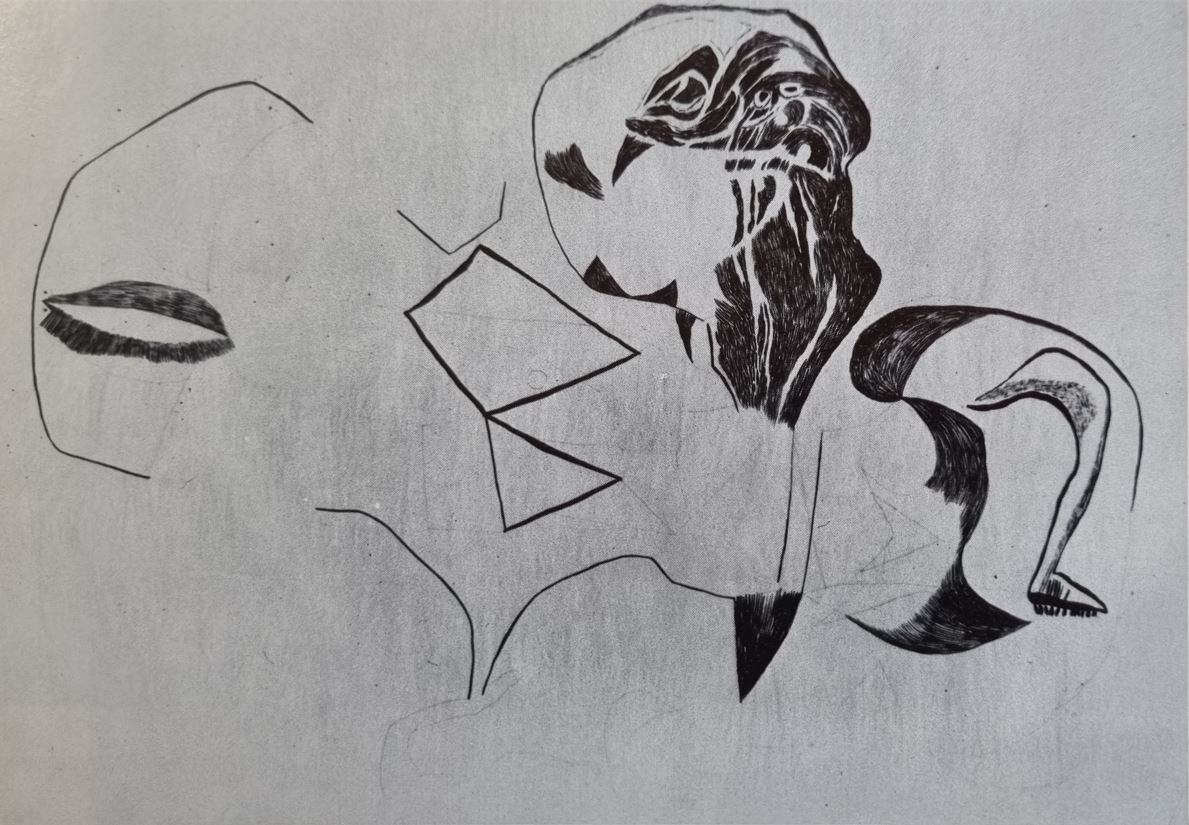This black and white impressionistic illustration features a predominantly white background with intricate and abstract linework throughout. On the left, a swirling, curling pattern seems to encircle one distinct element—a pair of lips—amidst the geometric designs, which include a couple of triangles and various circular shapes, both solid and empty. In the middle, there are geometric shapes: a diamond and a triangle touching at their corners. The central portion of the image hints at an impressionistic human face, albeit without distinct features like eyes, ears, or a nose, save for the lips on the far left. The area also exhibits a "hairish" circular motif, surrounded by swirling dark lines and shaded patterns that evoke a sense of depth and mystery. The right side of the image is filled with abstract outlines and organic, ornate textures, featuring curved and circular patterns that create a dynamic play of form and space. Overall, this illustration borders on the abstract and surreal, inviting each viewer to discern their own patterns and meanings from its complex interplay of lines and shapes.